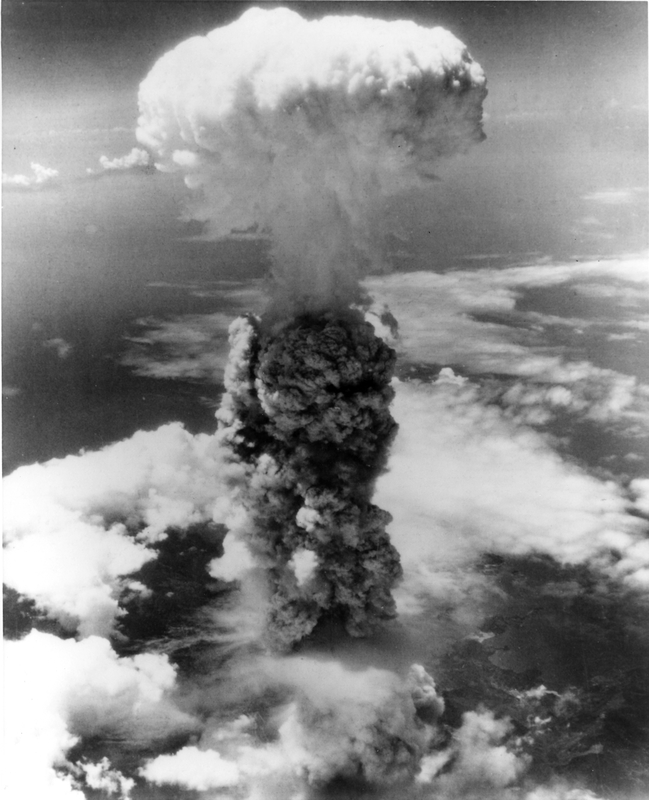This black and white photograph captures a dramatic mushroom cloud from a nuclear explosion, likely a historical test from around the World War II era. The image, taken from high in the atmosphere, reveals a massive plume piercing through a layer of regular clouds, with the ocean visible far below. The mushroom cloud, typical of fission bomb explosions, rises from a dark gray column of smoke that thins as it ascends before spreading out into a lighter gray, rounded "mushroom cap" at the top. The photograph is in portrait orientation, emphasizing the vertical expanse of the explosion against the backdrop of the sky.